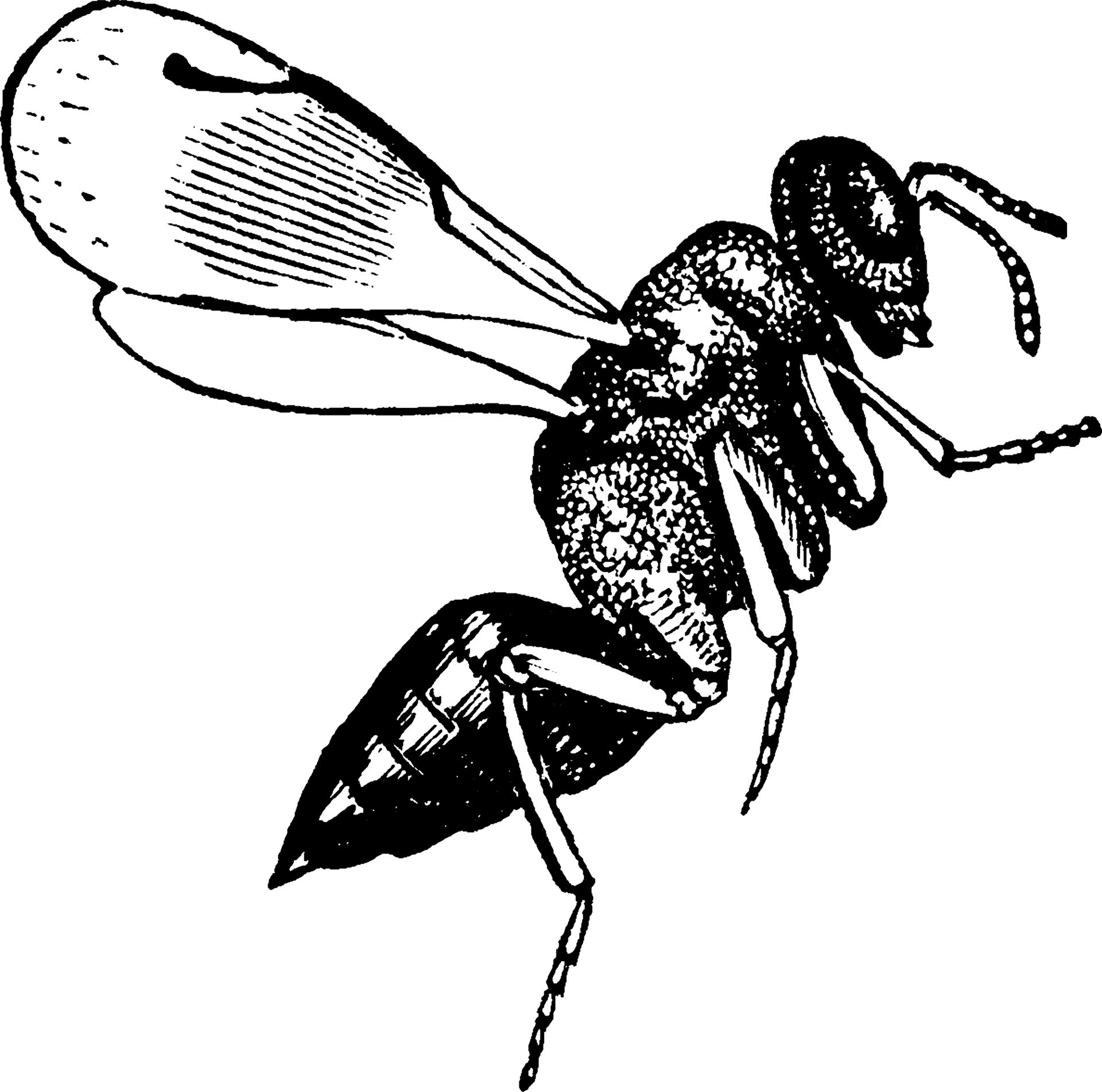This detailed black and white image appears to be a highly detailed sketch of a wasp. The wasp’s body shows complex detailing, with a predominant black coloration interspersed with white spots. Its tail, tapering to a sharp stinger shaded mostly in black, adds to the intricate illustration.

The wings of the wasp are primarily white but crisscrossed with fine black lines outlining their fibers, with a larger wing on top and a smaller one tucked behind it. The wasp's head is oval-shaped, exhibiting two downturned antennas and large, dark eyes outlined in black, though the facial features are somewhat indistinct.

Three of the wasp’s legs are visible; the two lower legs are oriented to the left while the upper leg stretches out to the right. The legs are white with black borders and have small spikes at their ends.

The combination of black and white shading throughout the wasp's segmented body, along with its distinct and detailed anatomical features, makes the image strikingly vivid despite being monochromatic.